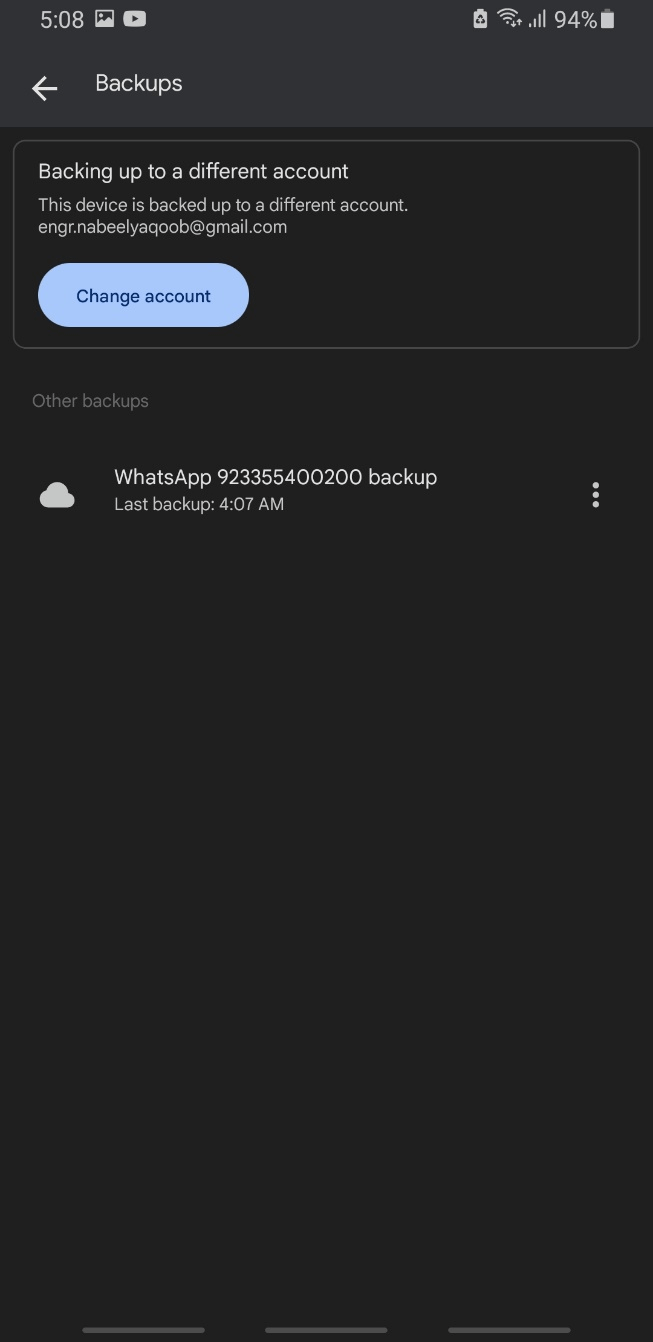Screenshot of a phone application interface:

- **Header Area (Dark Gray Background):**
  - **Time:** 5:08 AM displayed at the top left.
  - **Icons (Left to Right):**
    - A white picture icon.
    - A white YouTube icon.
  - **Top Right Status Indicators:**
    - Full battery symbol showing 94% charge.
    - Five signal bars indicating strong network connectivity.
    - Wi-Fi symbol indicating a connected Wi-Fi network.
    - Power-saving mode symbol in white.

- **Sub-header:**
  - The word "Backups" at the bottom of the dark gray bar.
  - A white arrow pointing left located beneath the word "Backups".

- **Main Content Area (Black Background):**
  - **Gray Rectangular Outline with Rounded Corners:**
    - **Title:** "Backing up to a different account."
    - **Description:** "This device is backed up to a different account."
    - **Listed Email Address**: Displays a personal email address beneath the description.
    - **Blue Button:** Labeled "Change Account".
    - **Subtext in Faded Gray:** "Other backups."
  
  - **Backup Item Listed:**
    - **Left Side Icon:** White cloud logo.
    - **Backup Details:** 
      - "WhatsApp, 923355400200, backup."
      - "Last backup, 4:07 AM."
    - **Additional Options:** Three vertical dots to the right for more options.

- **Footer Area:**
  - **Three Dark Gray Rectangles (Pill-shaped):**
    - Placed at the very bottom of the page.
    - Separated by a large empty area of the black background.

This detailed caption provides a clear and comprehensive description of the visual elements and layout within the screenshot of the phone application.